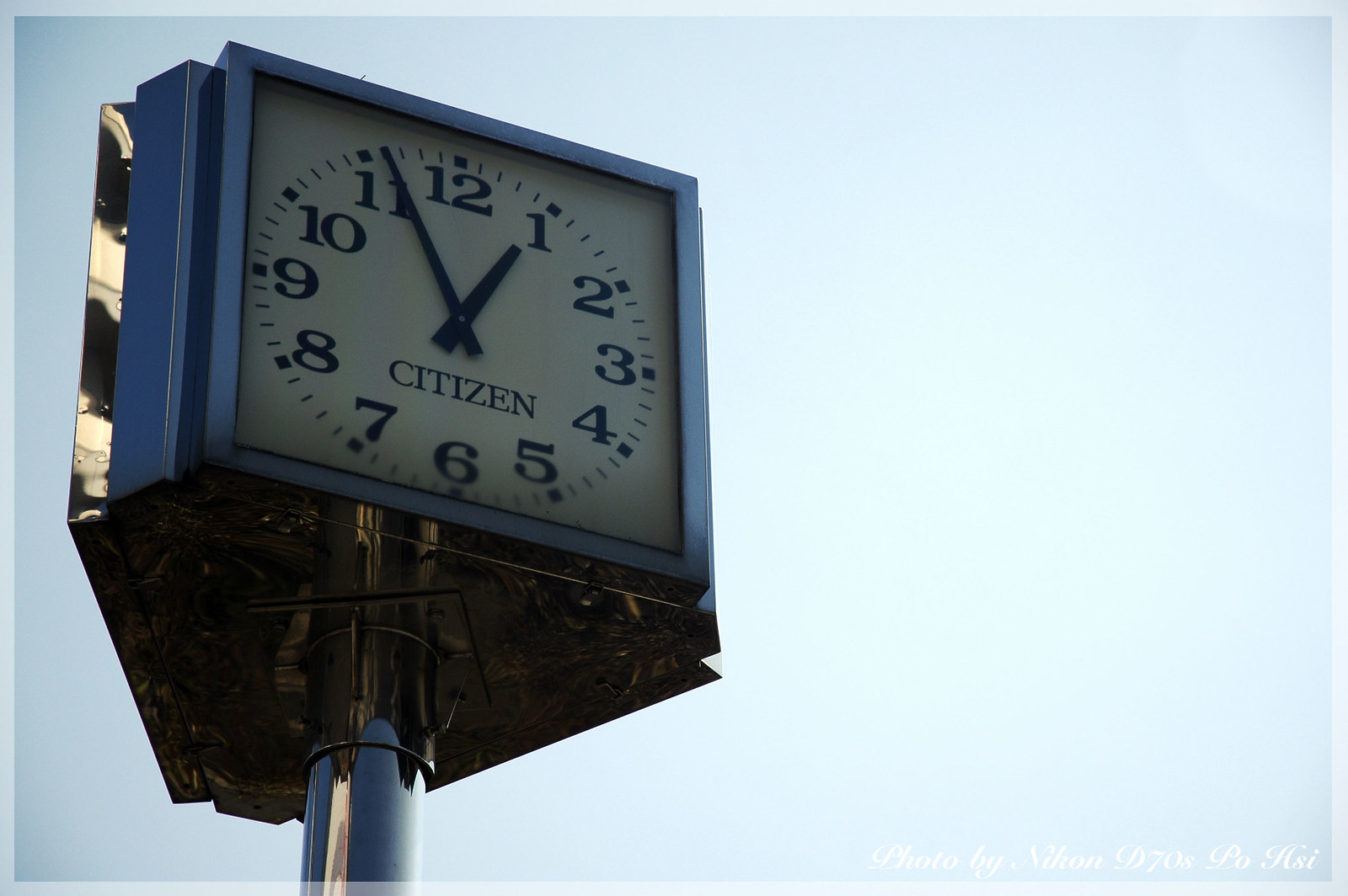A prominent Citizen clock is mounted atop a silver pole, which mirrors the blue hue of the clear sky, giving it a harmonious appearance. The clock face, which is square, stands out against the triangular underside of the mounting structure. The clock face is crisp white, adorned with bold black numerals, hands, and the distinctive Citizen logo, creating a sharp contrast that makes it easy to read. The time displayed is approximately 12:56.